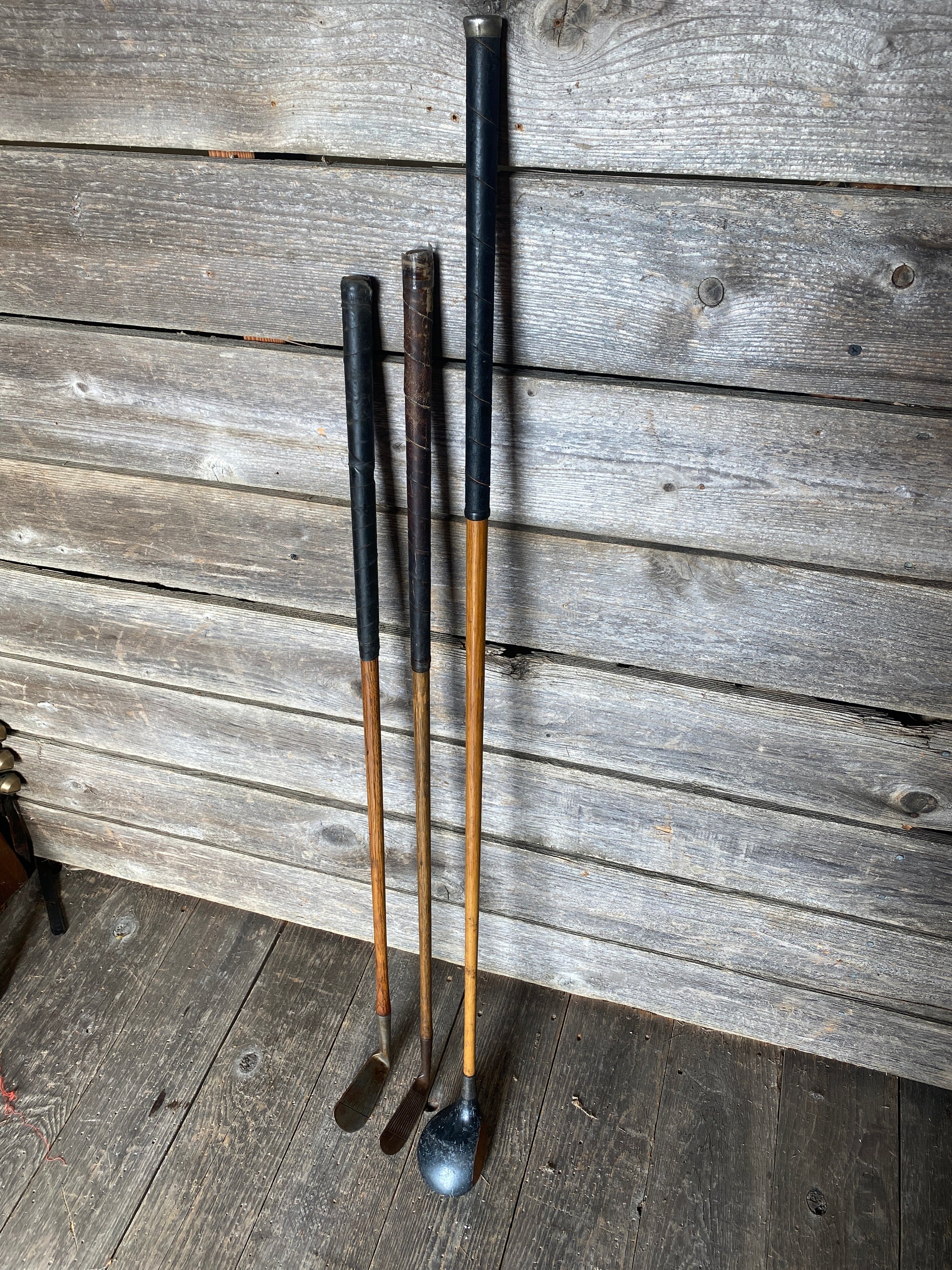This photograph, taken indoors, showcases three golf clubs positioned side by side against a wooden wall. Each club features a brown wooden shaft with a handle wrapped in either dark blue or brown material. The base portions of the clubs vary in shape and design. The setting resembles a wooden shed, characterized by wooden planks forming the wall and a floor with various shades of grey. The overall ambiance is rustic, emphasized by the natural wooden textures and the orderly placement of the golf clubs.